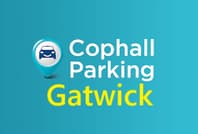The image is a slightly blurred, rectangular media graphic with a gradient blue background that transitions from a darker blue on the left to a lighter blue on the right. Centered in the middle of the graphic is the text "Cop Hall Parking," with "Cop Hall" positioned above "Parking" and both words in white. To the left of this text appears an icon that resembles an upside-down raindrop containing a circle, beside a small, blue cartoonish car with two eyes and a smile. Below the main text, the word "Gatwick" is displayed in a slightly larger, highlighted yellow font. Despite the blurriness, the overall content remains legible.